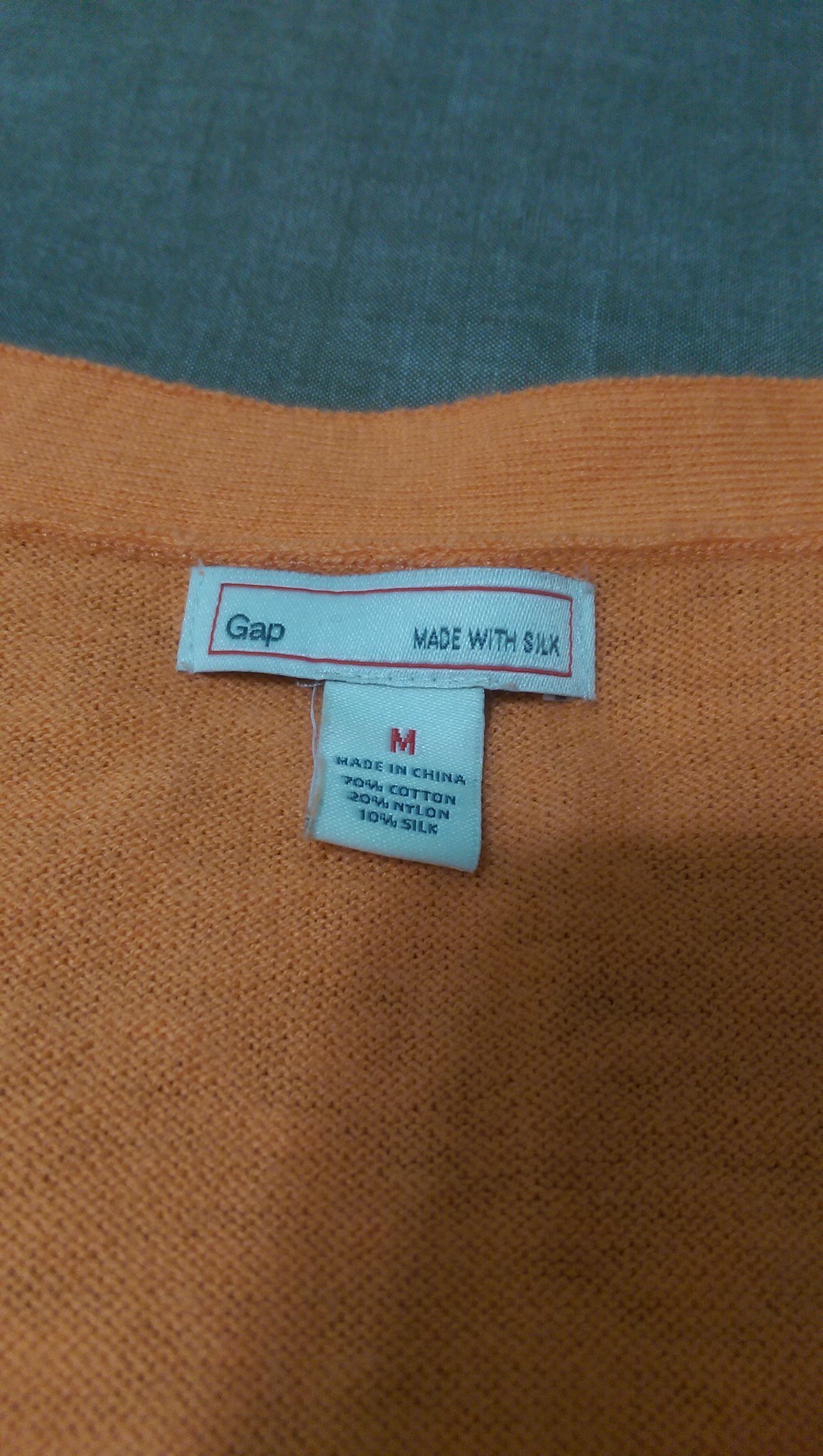This photograph features an old T-shirt of a burnt orange hue, fashioned from a material that resembles cable knit but is actually silk, as indicated by the tag. It is laid out against a denim backdrop. The T-shirt is a product of the brand GAP, as shown by the brand tag. Below the brand name, the label specifies the fabric composition as 100% silk and confirms that the item is a medium size. The tag is square with a conspicuous red "M". There is additional text, likely stating "Made in China," although it is somewhat blurred and diminutive, making it difficult to decipher.